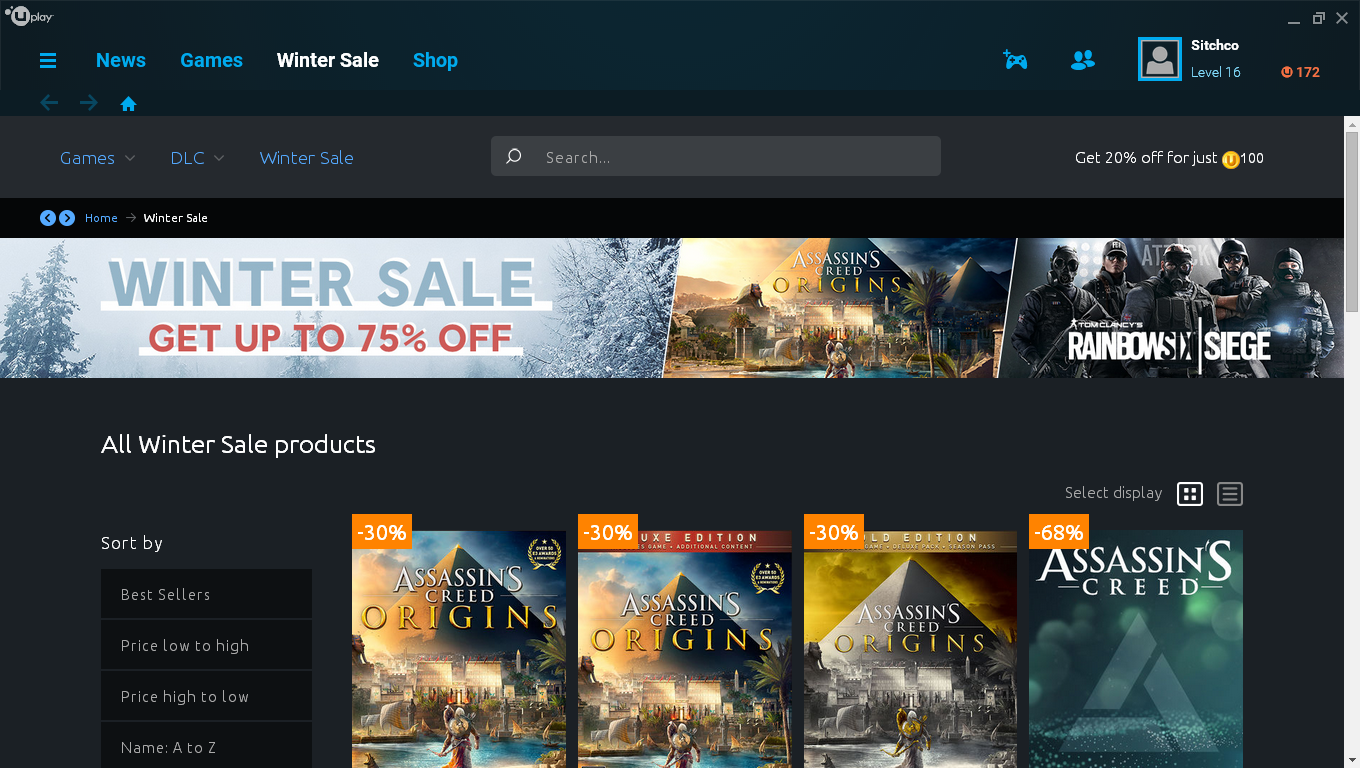The image showcases a website in dark mode with a focus on a winter sale section. The entire background is dark grey, providing a sleek and modern appearance. At the top of the interface, a navigation bar features menu options in blue text: the standard hamburger menu icon for additional navigation, followed by "News," "Games," and "Shop." The "Winter Sale" section is highlighted in white to indicate the current page.

To the far right of the navigation bar, an account section is visible, displaying the user's profile icon encased in a blue square. Beside it, the user’s name and account level (16) are also shown.

Directly below this top navigation bar, an additional menu appears, featuring options in blue text for "Games," "DLC," and "Winter Sale," accompanied by a search field. Next to the search field, a promotional note reads, "Get 20% off just for just a hundred."

A prominent banner beneath this displays "Winter Sale" with an eye-catching “Get up to 75% off” message. Accompanied by thumbnail images of popular games like "Assassin's Creed" and "Rainbow Six Siege," the banner also prompts users to explore "All Winter Sale Products" in bold white text.

On the left side, a sorting pane offers filtering options: "Sort by," "Bestsellers," "Price: Low to High," "Price: High to Low," and "Name: A to Z." The main content area below showcases four game titles available at discounted prices: "Assassin's Creed Origins" listed three times each with a 30% discount, and an original "Assassin's Creed" game with a striking 68% discount.